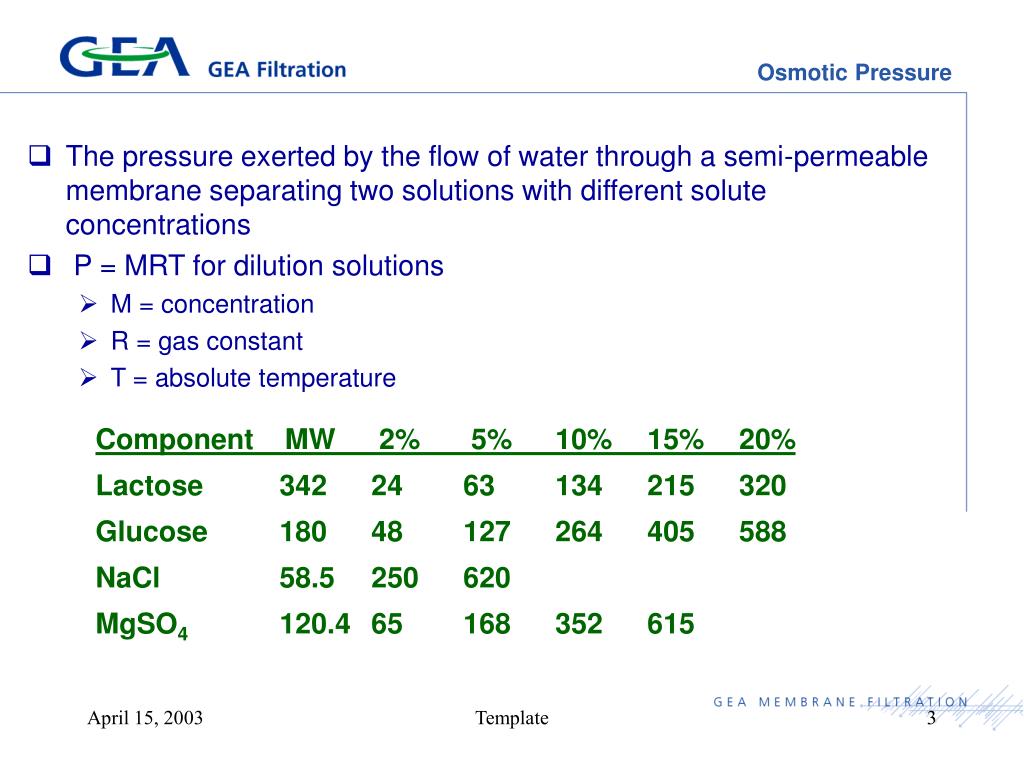The image depicts a horizontal rectangular chart focusing on osmotic pressure, marked on the right side. The top part features "GEA" in large capital letters with "GEA Filtration" in smaller text, all accented by a green halo. A thin blue border runs along the top and right sides.

Below "Osmotic Pressure," the chart provides two bullet points in blue text within white squares outlined in blue. The first bullet point, spread over three lines, explains, "The pressure exerted by the flow of water through a semi-permeable membrane separating two solutions with different solute concentrations." The second bullet point states the formula, "P = MRT for dilution solutions," with sub bullets detailing the variables: "M = concentration," "R = gas constant," and "T = absolute temperature."

Underneath these points, a table in green text lists components alongside their respective molecular weights (MW) and various concentration percentages (2%, 5%, 10%, 15%, 20%). The components listed are lactose, glucose, NaCl, and MgSO4. The lower-left corner of the page notes the date "April 15, 2003," and the middle bottom mentions "template." The entire chart is set against a white background.